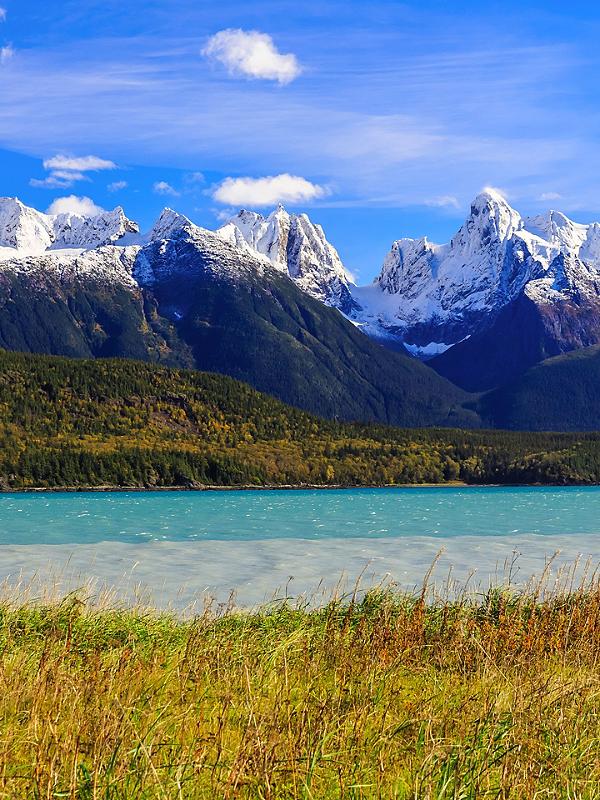This photograph captures a stunning, snow-capped mountain range with a mix of jagged peaks prominently displayed in the foreground. The sky overhead is an incredibly vivid blue, sprinkled with a few wispy cirrus clouds predominately to one side of the image. Below the mountain range, there's a hilly area lush with a variety of green tree cover, ranging from dark to tannish green, indicating the robust diversity of the forest. Nestled at the base of the hills, a crystal-clear, vibrant blue mountain lake stretches across the scene. The water's edge on the far side subtly transitions to a more whitish hue, perhaps indicating the presence of frozen ice or sand beneath the surface. In the very foreground, the image is framed by a meadow of long, native grasses that are shades of green and brown, completing this picturesque landscape that seamlessly transitions from the serene, grassy forefront to the cold, imposing beauty of the snowy mountains in the distance.